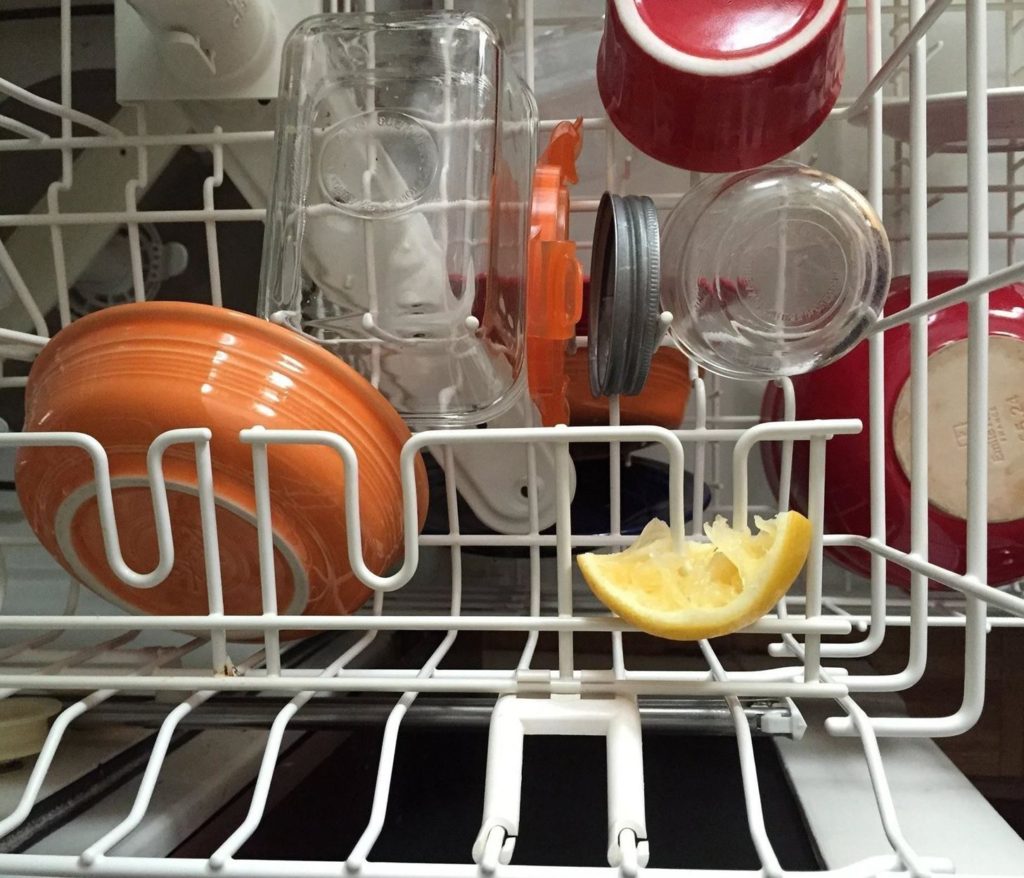Caption: 

The image provides a detailed top-down view into the interior of a dishwasher. The white, rubber-coated racks that hold the dishes form the background, creating a stark contrast against the various utensils and containers. At the top center, the underside of the water-spraying arms is visible, hinting at the mechanics of the appliance.

Prominently displayed is a red casserole dish with a white rim around its top, positioned near the middle. Adjacent to the casserole dish is a clear glass baking dish. An orange item, likely a lid, adds a splash of color beside the baking dish. A grayish-black jar lid is seen near a glass jar, indicating a scattered assortment of kitchen items.

Toward the bottom right, a red bowl with a distinctive white base stands out. Next to it lies a used lemon, squeezed and abandoned. To the left of the lemon, an orange bowl completes the colorful array. Beneath the racks and dishes, a black space marks what might be the door of the dishwasher, currently out of sight.